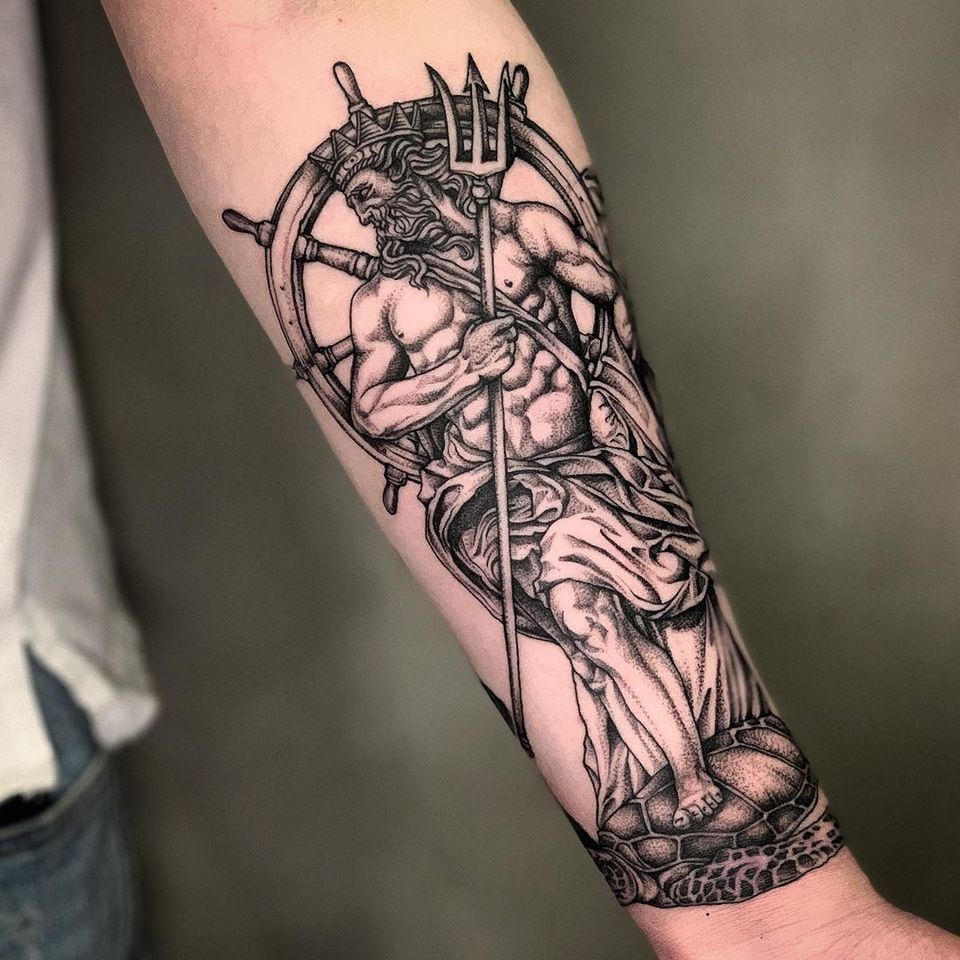The image showcases the inner forearm of a man dressed in a white top and blue denim bottoms, featuring a large, freshly-inked tattoo that spans from the wrist to the elbow. The detailed black ink design portrays Poseidon, the Greek god of the sea. Poseidon, a muscular figure with a crown, long flowing hair, and a beard, is depicted standing amid a ship's captain wheel. He is shirtless, wearing a robe that drapes from his waist down to his knees and a sash over his shoulder. In one hand, he wields a trident, while his other arm rests behind the robe. His foot is planted on a sea turtle, giving the impression he is floating above it. Surrounded by slight redness that hints at the tattoo's recent application, Poseidon's gaze is directed leftwards, adding a dynamic sense of character to the intricate body art.